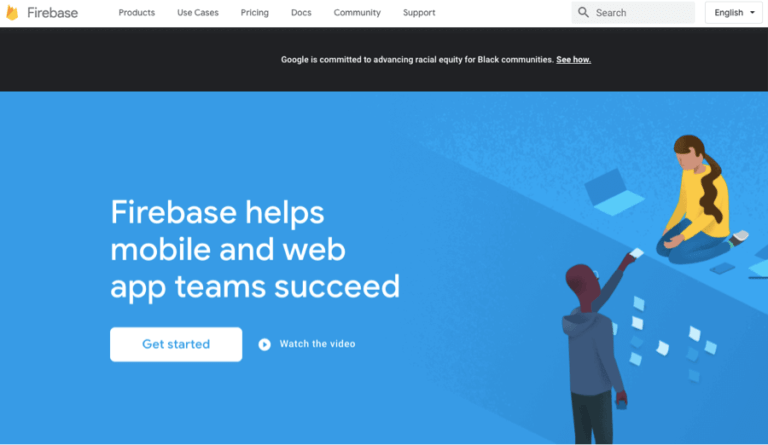A screenshot from a website featuring the Firebase platform is prominently displayed. The background of the website is illustrated in a cartoonish, clip-art style with a predominantly blue color scheme and a black banner at the top. In the middle-left section of the page, large white font reads: "Firebase helps mobile and web app teams succeed." 

On the top left corner, the Firebase logo is visible, featuring gray lettering with an orange and yellow flame emblem to the left. The central cartoon image depicts a bald, black man wearing a blue-gray hoodie, black pants or jeans, and glasses. He is handing a small square piece of white paper to a woman situated on a higher ledge. The woman, drawn in the same cartoon style, has a long brown ponytail, a yellow long-sleeve shirt, and jeans. Although both characters lack detailed facial features, their interaction is clear as the woman has her hand outstretched to receive the paper. A laptop is positioned next to her on the ledge, emphasizing the tech-focused theme of the scene.